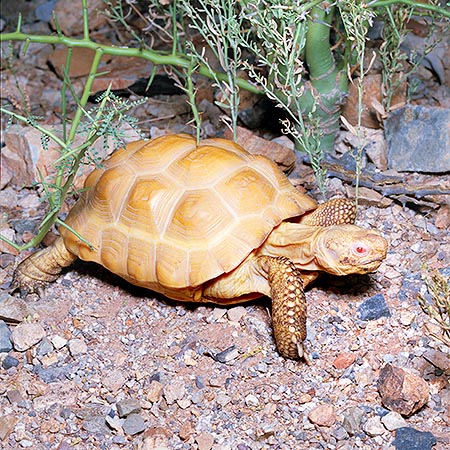The photograph captures a detailed scene of a tortoise in its habitat, likely a terrarium that mimics a desert or warm climate. The tortoise, with its textured, scalloped shell in shades of light and dark brown, is moving from left to right. The shell is characterized by numerous bumps, adding to its rugged appearance. The tortoise's skin is a beige flesh color, with a rough, leathery texture reminiscent of alligator skin, and its legs are splayed out as if in mid-motion. The tortoise’s eyes are a striking red. 

The background is filled with an assortment of vegetation, including green leaves and branches, some of which appear spiky. Rocks of varying sizes and colors—beige, grey, and bluish-grey—are scattered throughout, creating a rocky and dry terrain. The ground is covered in small, gravel-like pebbles. The setting is completed with a mix of leaf debris and grass. The overall color palette of the image includes a blend of brown, beige, green, grey, and subtle hints of blue, orange, white, and black, providing a realistic and earthy depiction of the tortoise in its carefully curated environment. The photograph is likely taken indoors, as the controlled setting suggests a pet habitat.